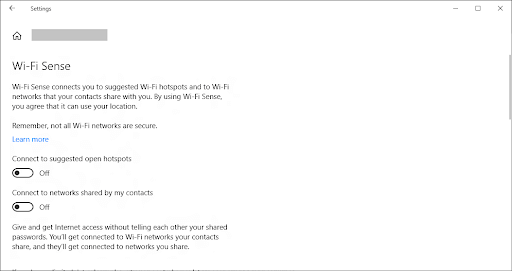The image serves as a screenshot of a Wi-Fi settings page with a white background and a black border. On the right side, the screen is mostly blank, with the exception of a black 'X' icon in the top right corner. To the left of the 'X', there is a black-outlined box with a white interior and a black minus sign inside. About two inches from the top right corner is a two-inch black, broad vertical border. 

On the left side of the image, starting from the top left corner, there is a left-pointing arrow labeled "Settings". Below that, there is a home icon followed by a gray search bar. Large lettering spells out "Wi-Fi sense (S-E-N-S-E)" beneath the search bar. Underneath this heading, three lines of information explain the feature:

- "Remember not all Wi-Fi networks are secure."
- "Learn more" (in blue text and likely a clickable link).

The status "Connected to suggested open hotspots" has a toggle switch next to it, currently in the "off" position. Below it, there’s another option stating "Connect to network shared by my contacts," also toggled off. The word "off" appears to the right of these switches.

The text at the bottom of the screenshot states: "Give and get internet access without sharing your passwords. You'll get connected to Wi-Fi networks your contacts share, and they'll get connected to the networks you share."